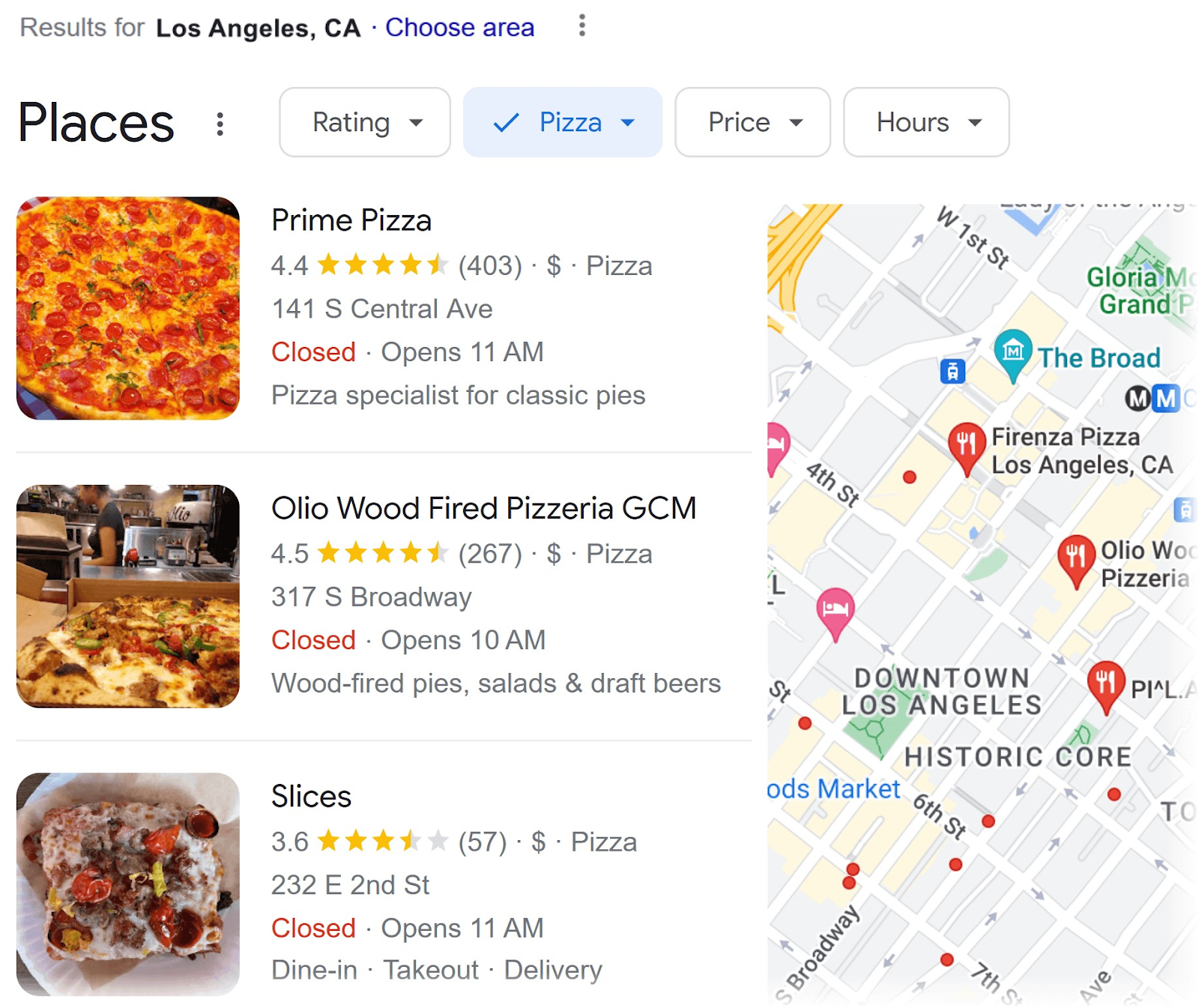Here's a detailed and cleaned-up caption for the given image:

---

The map of Los Angeles, California on the right highlights several pizza places along with other landmarks such as a church and a gas station. Featured prominently are three top-rated pizza restaurants:

1. **Prime Pizza**: Located on Central Avenue, Prime Pizza has a 4.4-star rating and is budget-friendly with a single dollar sign. Although currently closed, it opens at 11 a.m. Known for its classic vibes, their specialty thin-crust pepperoni pizza is light on cheese but loaded with flavor.

2. **Olio Wood Fired Pizzeria**: Boasting a 4.5-star rating and also marked with one dollar sign, Olio Wood Fired Pizzeria is highly praised. This establishment offers wood-fired pies, salads, and draft beers. Though closed at present, it reopens at 10 a.m. Their pizzas are known for a generous amount of cheese, making it the standout choice among the featured eateries.

3. **Slices**: Found on East 20th Street, Slices has a 3.6-star rating from 57 reviews with the same one dollar sign. It is currently closed but will open at 11 a.m. The restaurant provides dine-in, take-out, and delivery options. However, its pizza appears less appealing compared to the others.

Overall, **Olio Wood Fired Pizzeria** emerges as the best-rated choice for cheesy, wood-fired pizzas in this selection.